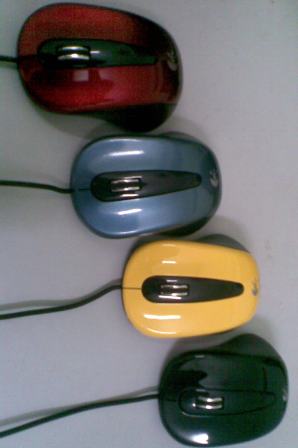This color photograph depicts four computer mice meticulously arranged in a descending diagonal line from the upper left to the lower right of a portrait-style rectangular frame. The background appears grey, despite some accounts suggesting a white surface, and casts slight shadows beneath the mice. Each mouse, identical in form except for their vibrant colors, boasts a distinctive black central strip and a matching scroll wheel with a black line down the middle.

The topmost mouse, positioned in the upper left corner, is striking in its rust-red hue and features a black midsection and scroll wheel. A small piece of cord protrudes behind it.

Directly beneath the red mouse, situated centrally in the image, is a steely blue mouse with a similar black central strip and scroll wheel. More of its black cord extends outward towards the left.

Following the blue mouse is a bright yellow one, also bearing the consistent black midsection and scroll wheel design. It has a noticeably longer cord emerging from its back.

The line concludes with a sleek black mouse positioned near the bottom right corner. Though its details blend more with its cord and background, it maintains the identical design seen in the other mice.

All mice are wired, facing to the left, and reflect light, particularly the blue one, highlighting their glossy surfaces. The prominence of the cords and uniformity in design reinforce the orderly arrangement and coherence of these computer accessories.